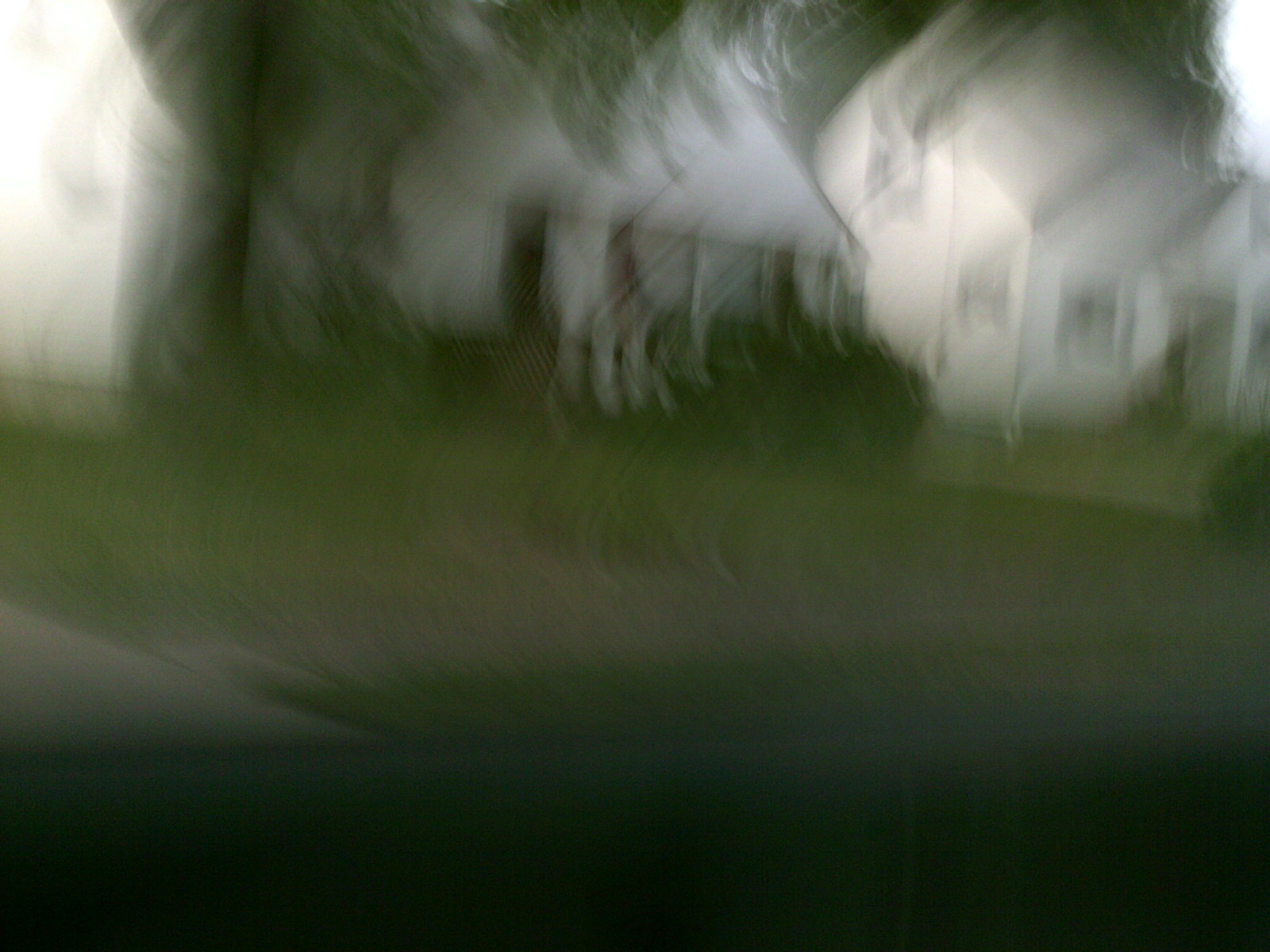A blurred image depicts a quiet residential street with three Cape Cod-style houses. The bottom of the picture is very dark, likely indicating the street, while patches of brown and green suggest yards and driveways. The houses are white with regularly pitched shingle roofs, also white, but the entire scene is veiled in a whispy, cloud-like blur that imparts a slightly gothic ambiance.